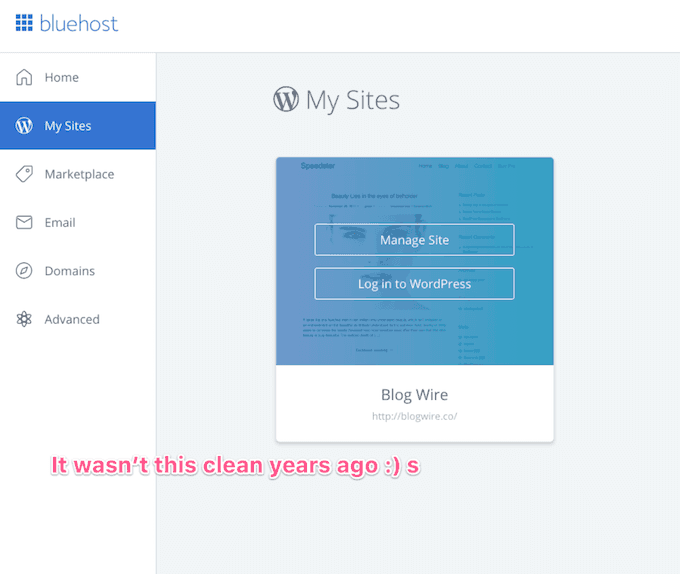The image is predominantly square, featuring a white background on the top and left side, transitioning to a light gray background on the remainder of the frame. In the top left corner, the word "Bluehost" is visible. Below this, in the white section, is a vertical navigation menu listing options such as Home, WordPress, My Sites, Marketplace, Email, Domains, and Advanced. The "My Sites" option is highlighted with a blue background.

To the right, against the light gray background, is the section titled "My Sites." Centrally located is a square window, where the top portion is slightly translucent, revealing part of the page underneath. This window has a light blue overlay with two stacked buttons labeled "Manage Site" and "Login to WordPress." At the bottom of this window, on a white background, the text "Blog Wire" is displayed. Superimposed at the very bottom, in pink text, it reads "It Wasn't This Clean Years Ago," accompanied by a smiley face emoji.